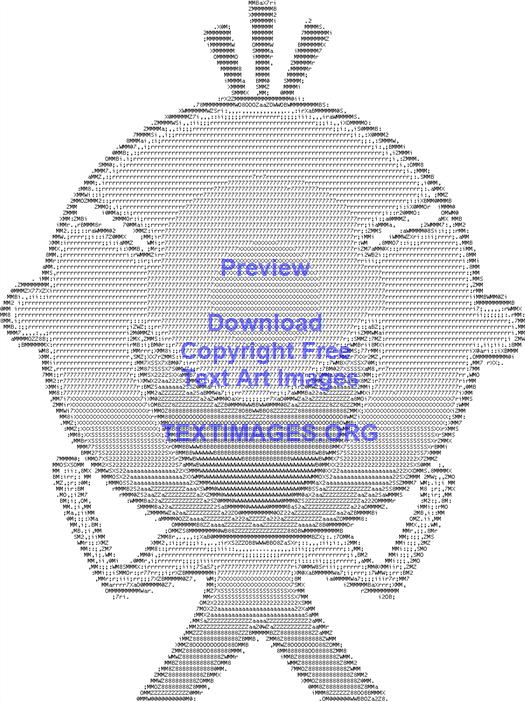The image is a digital screenshot of a cartoonish clip art character, available for purchase online, as indicated by the blue watermark in the center reading "preview, download, copyright free, text art images, textimages.org." The character, possibly depicting a little boy or a small man, has an overly large round head, small slanty white slits for eyes, and three black strands of hair on top. The character is standing with its legs apart and arms raised to the sides in a power pose, resembling someone flexing their biceps. The entire figure displays a printed design with dark and light bluish speckled patterns, except for the eyes which are plain white. The body is roughly half the size of the head.